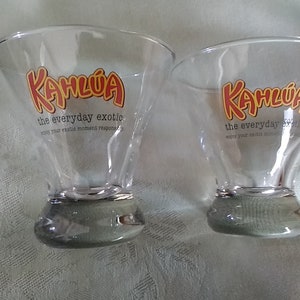This color photograph features two shot glasses laying on their sides on a white tablecloth, bathed in ample lighting, likely taken in a home or bar setting. The shot glasses are identical and display large red letters outlined in yellow that spell out "Kahlua." Below this, the text reads "The Everyday Exotic," followed by some smaller, unreadable text with the word "Your" distinguishable among the verbiage. The glasses have a greyed bottom due to the transparency interacting with the fabric underneath. The shot glasses possess a narrow base and a wide opening, characteristic of typical shot glasses. Kahlua, a sweet, flavored liqueur often consumed in mixed drinks, is highlighted on the front of both glasses.